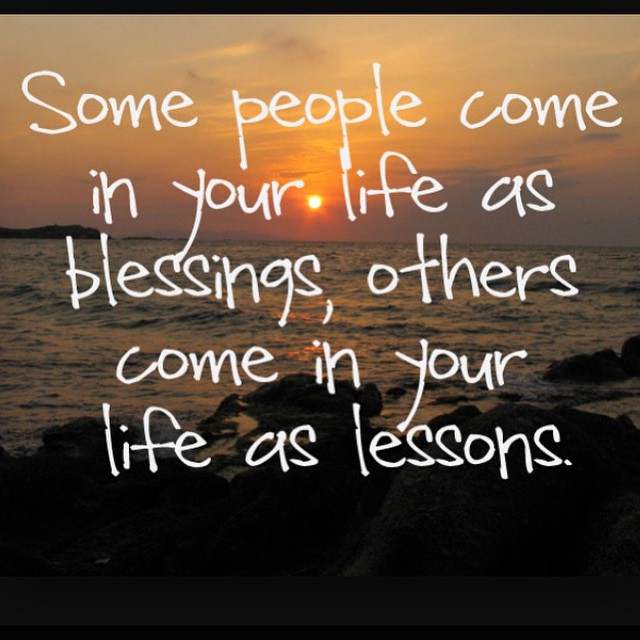The image is a dark, visually striking photograph of a rocky shoreline at sunset, with a thin black border at the top and bottom. The foreground features dark rocks and slightly choppy ocean waves lapping the shore. The horizon reveals the orange sun low over the water, casting an intricate reflection and painting the sky with a blend of orange, purple, and blue hues. Above the scene, white text appears in a cursive-like font, likely added through digital editing, with the inspirational message: "Some people come in your life as blessings. Others come in your life as lessons." The photo lacks any human presence, focusing purely on the serene and evocative natural landscape.